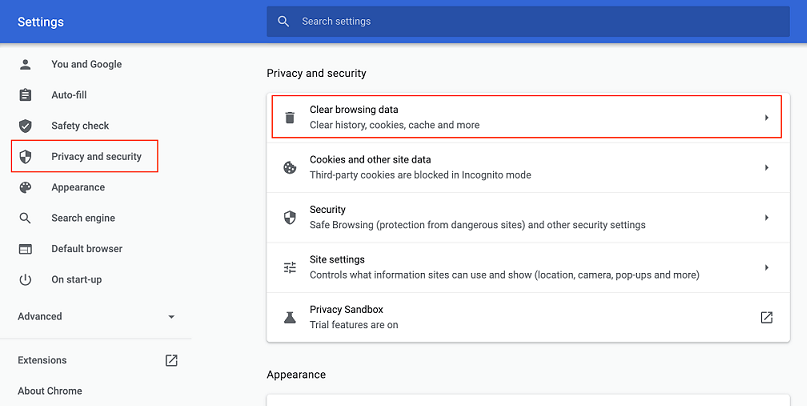In this detailed image, we see a screenshot of the Chrome browser settings interface. The interface features several sections listed prominently on the screen:

1. **Settings Overview**: This is the initial view where various options are visible.
2. **Search Settings**: A section dedicated to customizing search preferences.
3. **Autofill**: Facilitates managing saved addresses, payment methods, and other autofill details.
4. **Privacy and Security**:
   - **Cookies and Other Site Data**: An area dedicated to managing site data and cookies, including third-party cookies.
   - **Safe Browsing and Security**: Options to enable safe browsing, protection of potentially harmful sites, and other security settings.
5. **Site Settings**: Allows users to control what information sites can access and display, such as location, camera access, and notifications.
6. **Appearance**: Enables customization, showing a predominantly white background with a notable blue bar at the top, alongside options for themes and other visual adjustments.
7. **Search Engines**: Preferences for setting default search engines.
8. **Default Browser and Startup**: Settings for managing the default browser and configuring startup behavior.
9. **Extensions**: Area to manage installed browser extensions.
10. **About Chrome**: Information about the current version of Chrome.

Various toggle controls and drop-down menus are visible, allowing for granular management of privacy, security, and appearance. The interface is user-friendly, depicted with symbols that illustrate people, squares, and rectangles to enhance understanding. The browser's layout reflects a clean, modern aesthetic, with functional sections clearly demarcated for ease of navigation.